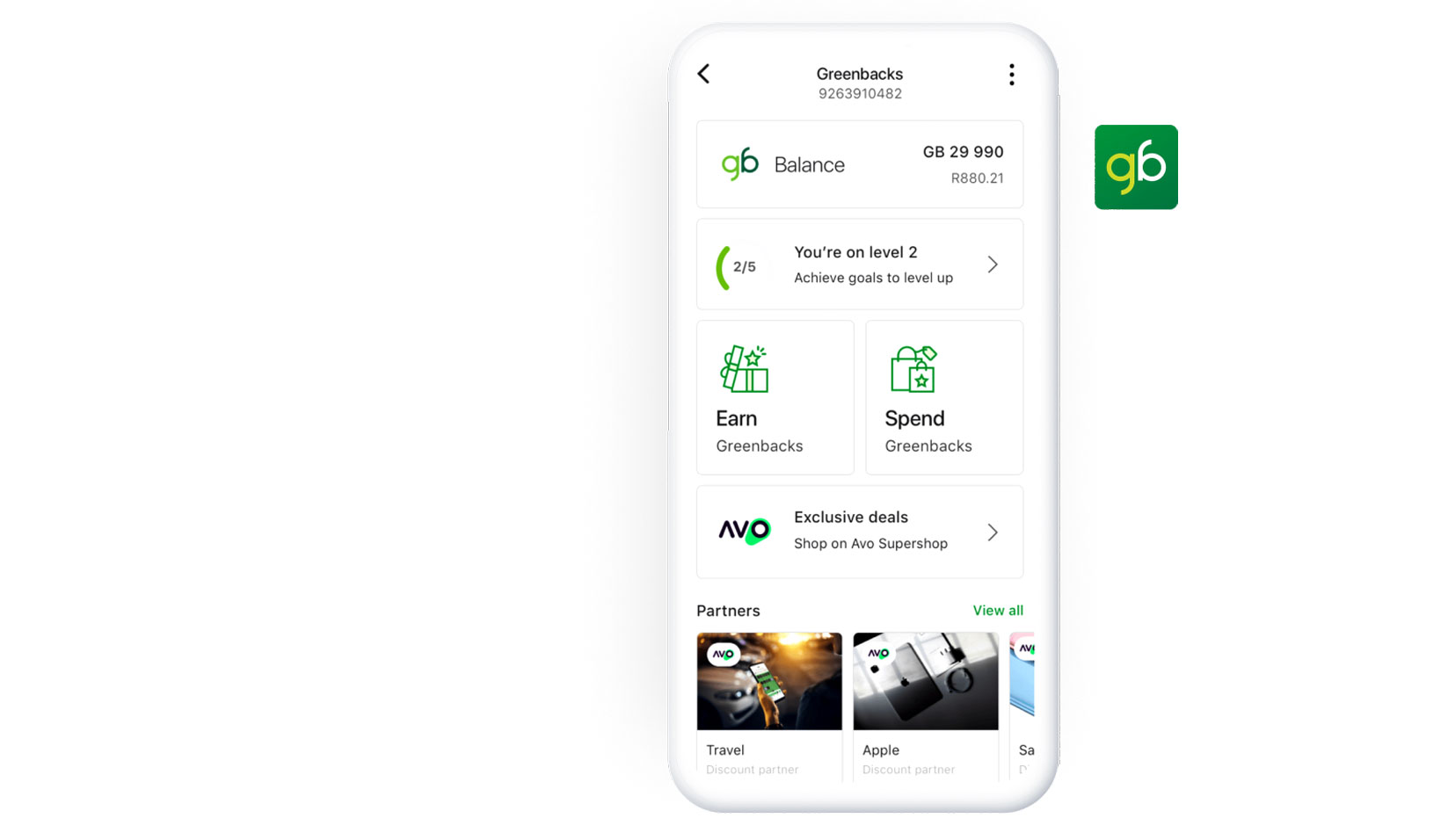This graphic presents an abstract representation of a smartphone with a simplistic design. The phone features a solid white color, with a white screen and bezels giving it a non-realistic appearance. It appears as though a fake screen has been photoshopped onto the front of the device. Adjacent to the smartphone on the right side of the image is a green square displaying a logo comprised of a yellow 'G' and a white 'B'.

On the smartphone screen, at the top in black font, the text "Greenbacks9263910482" is displayed. To the left of this text, there is an arrow pointing left, and to the right, there are three vertical dots. Directly below this header, a black outlined rectangle contains the text "GB Balance GB29990R880.21." 

Underneath this balance information, another rectangle includes the message "You're on level 2 out of 5. Achieve goals to level up." An arrow pointing to the right accompanies this message. Further down, two squares are displayed side-by-side. One square reads "Earn Greenbacks," while the other square states "Spend Greenbacks."